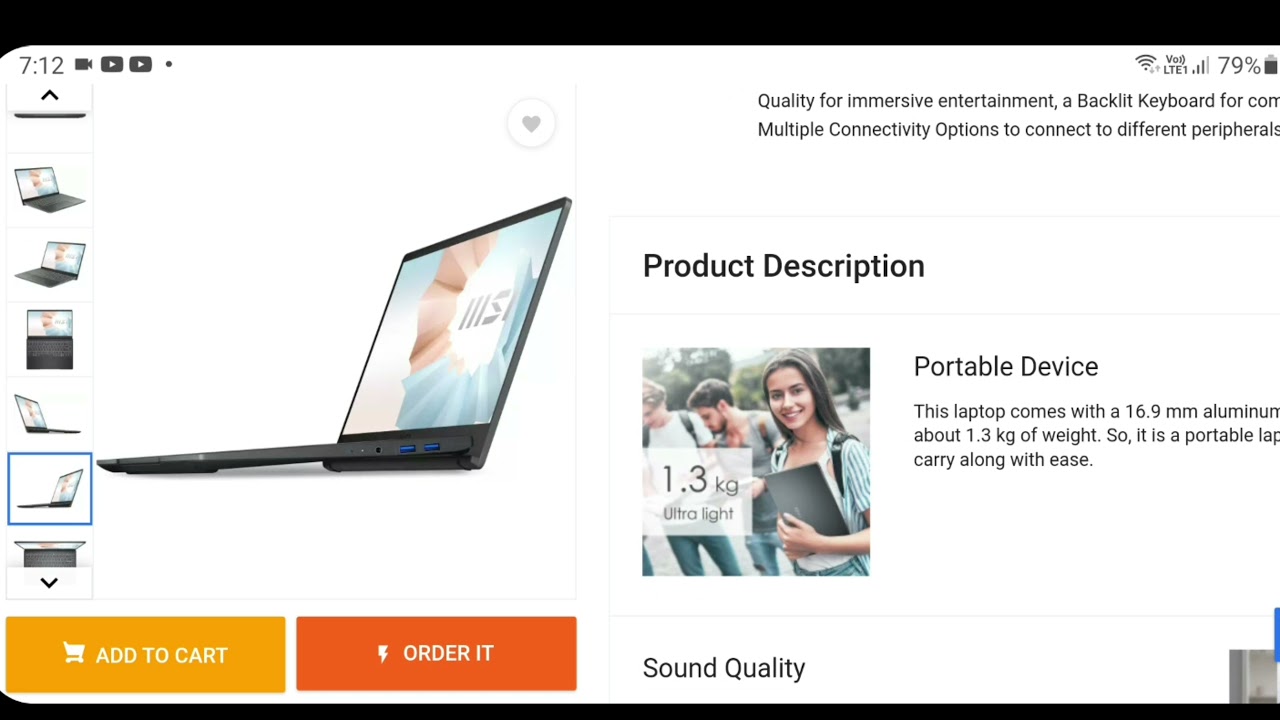The screenshot displays a predominantly white webpage with a clean layout and several sections. At the top of the page, a black bar spans across the width, housing various icons. The left side features the time, a camera icon, and two play buttons distinguished by black backgrounds with white arrows. To the right, icons for Wi-Fi and battery levels are present.

Below the time on the left, there is a drop-down menu indicated by a caret. This vertical column contains six smaller images, each depicting different views of a laptop. These variations show the laptop in various positions, including an aerial view, side profiles, and as flat.

Adjacent to this column is a larger image of the laptop, prominently displayed, with text highlighting some of its key features. One of the key points emphasizes the device’s portability, describing it as ultralight at 1.3 kilograms and having a sleek 16.9 millimeter aluminum body. Another photo below features two or three individuals, one of whom is holding the laptop, further emphasizing its lightweight nature.

Further down the page, there are interactive buttons for purchasing options: a yellow "Add to Cart" button and a red "Order" button. The section concludes with a mention of "sound quality," though the details are partially obscured.